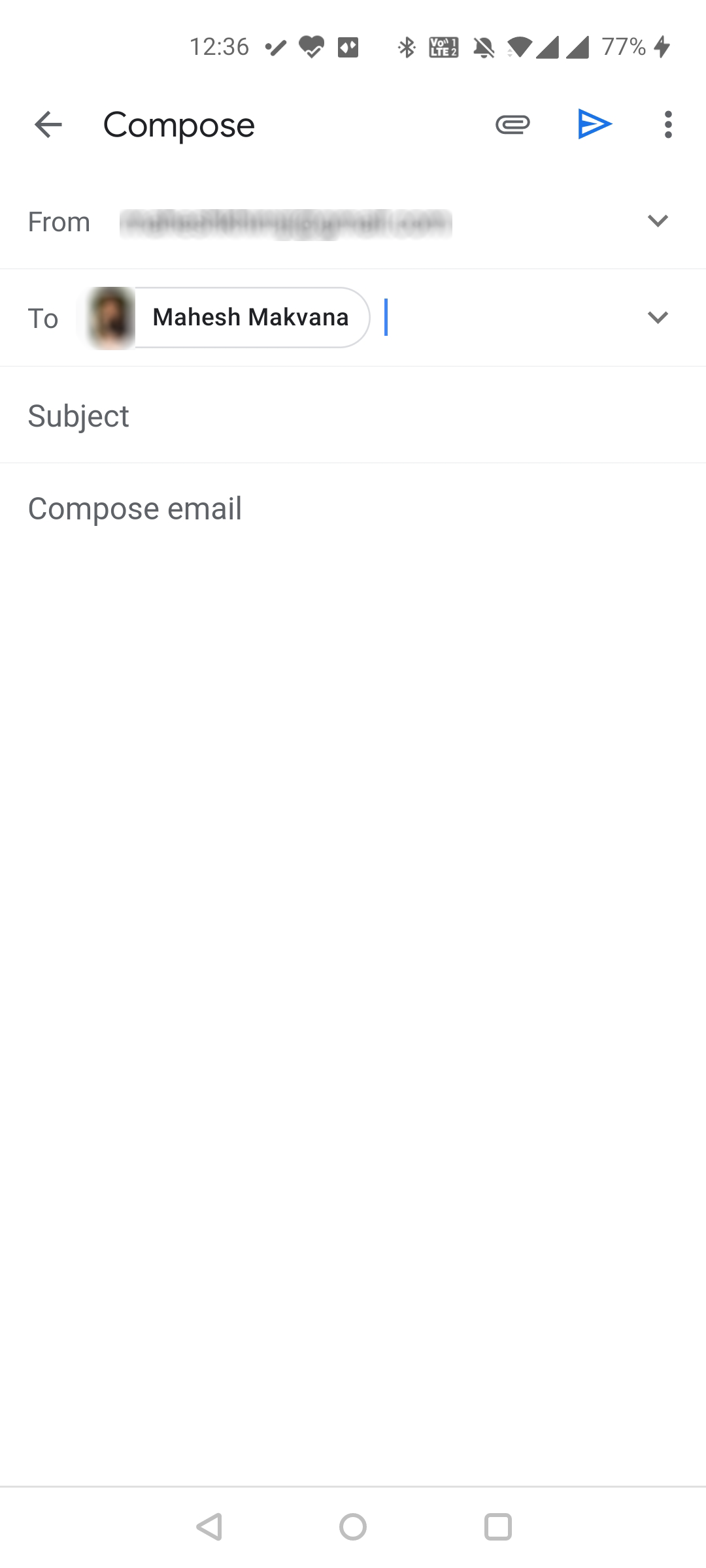In this detailed image, we observe a screenshot of an email displayed on a smartphone, likely an Android device. The background of the screenshot is entirely white, providing a clean visual for the email content. At the very top of the screen, several status icons are visible, including the battery percentage, which is at 77%, the Wi-Fi connection symbol, a heart icon, a Bluetooth symbol, and the current time, 12:36. 

Below these icons, there is a text field with the label "Compose" and an arrow on the left side indicating a back function. The "From" field contains a blurred-out name, maintaining confidentiality, while the "To" field shows an avatar of a person named Mahesh Makbana. Both the "From" and "To" fields have adjacent double arrow icons, suggesting expandable or interactive elements. 

In the body of the email, there is a subject line present, accompanied by a "Compose Mail" icon, indicating the process of drafting a new email. At the bottom of the screen, the standard Android navigation buttons are displayed: a triangle pointing left for the "Back" function, a circle for the "Home" button, and a square for the "Recent Apps" function.